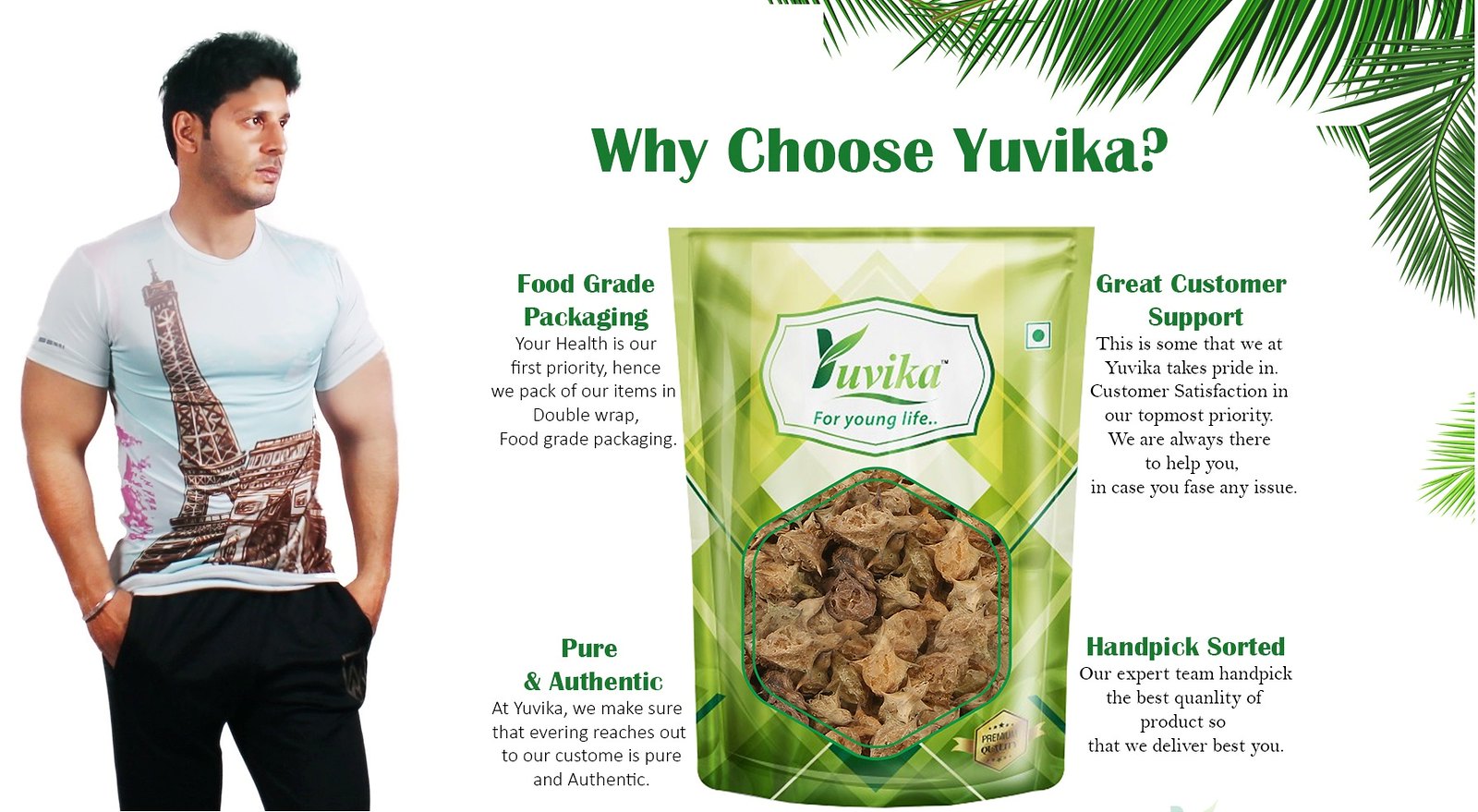In this advertisement for a product called "UVIKA," set against an all-white background, an Indian or possibly Hispanic man is depicted on the left side. The man, shown either as a digital rendition or a photographed individual, has dark hair and a stern expression. He is dressed in a white shirt featuring an Eiffel Tower design, black jeans, and has his hands in his pockets while looking towards the advertisement. The ad features a green package prominently placed in the center, labeled "UVIKA for young life." The package's contents are not clearly visible but suggest it may be a natural snack or supplement.

Surrounding the central package, various text blocks emphasize the product's benefits: "Why choose UVIKA?" "Food grade packaging," "Pure and authentic," "Great customer support," and "Hand-picked, sorted." The background includes some green palm or fern leaves in the upper right corner, adding a natural touch. The overall color scheme includes white, black, tan, light blue, brown, pink, green, and light green, enhancing the natural and healthy appeal of the product.